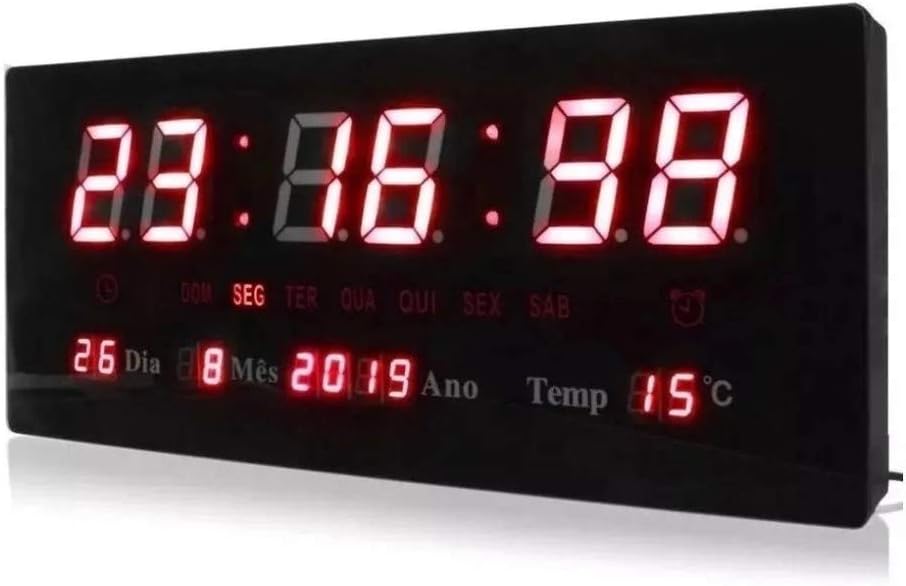This close-up image showcases a sleek, black digital clock set against a dark background. The clock displays the time in military format with red, glowing LED digits showing "23:16:98," indicating 11:16 p.m. It also features a detailed date and temperature display in both Spanish and English. The date line reads "26 DIA, 8 MES, 2019 ANNO" in Spanish, translating to the 26th day of the 8th month, 2019. Besides the date, the temperature is given as 15 degrees Celsius. The device has a slim, 3D rectangular shape and appears to have a small cord protruding slightly from the right side, extending out of the image frame. The close-up nature of the photo provides an intimate view of the clock's details but leaves the surrounding environment unseen.